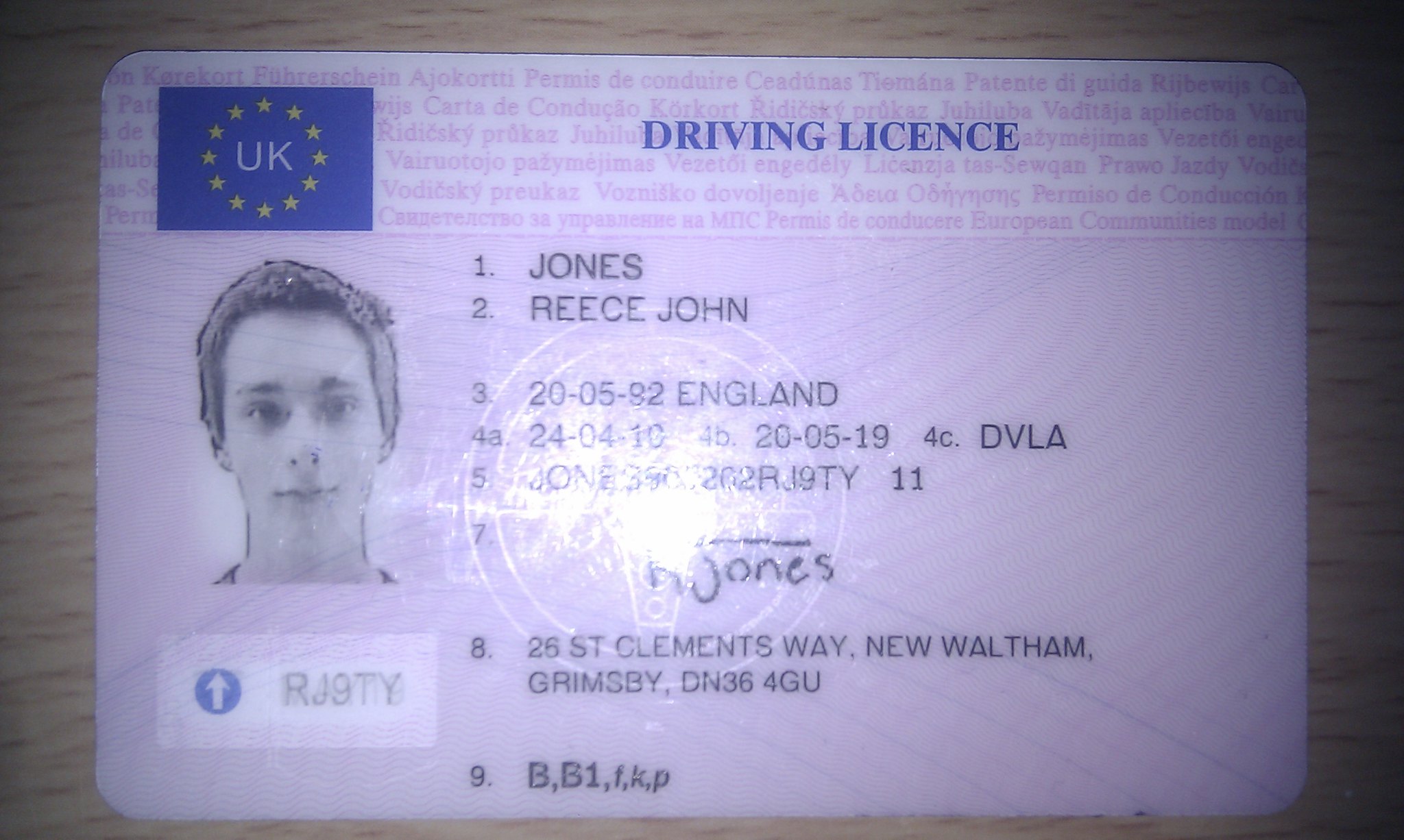The image is a detailed photograph of a United Kingdom driving license, set against a predominately white backdrop adorned with intricate purple and blue watermark designs. In the top left corner, a blue rectangle with a circle of stars surrounds the white text "UK." Centrally positioned at the top, the text "DRIVING LICENSE" is displayed in blue. Dominating the lower middle section is a photograph of an individual looking straight ahead, positioned towards the left center of the license. To the right of the photograph, there are several lines of black text providing personal information: 

1. Last Name: Jones
2. First Name(s): Reese, John
3. Date of Birth: 20/05/92, England
4A. Valid From: 24/04/10
4B. Valid To: 20/05/19
4C. Issuing Authority: DVLA
5. (Repeatedly stated: Last Name: Jones)
8. Address: 26 St. Clements Way, New Waltham, Grimsby, DN36 4GU
9. Additional Codes: BB1 FKP, RJ9 TY.

Due to the reflection from a light source, some portions of the text are illegible. The overall composition of the image is horizontal, centering on the ID card itself, with various colors such as blue, yellow, white, black, and gray contributing to the design.